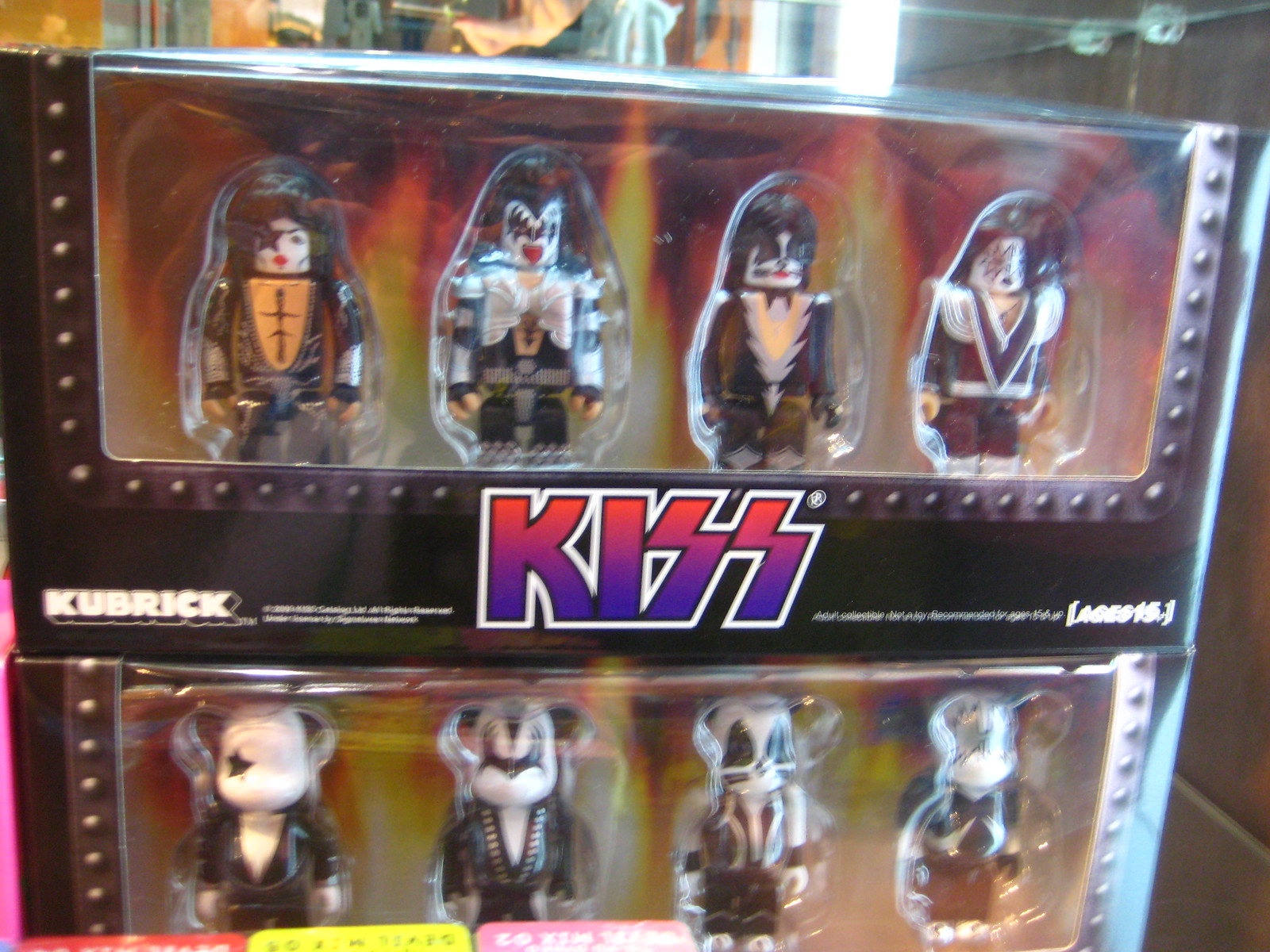The image depicts a packaged set of collectible toy figures representing the iconic rock band KISS. The package contains a total of eight figures arranged in two rows, with the top row featuring four Lego-styled miniature figures and the bottom row showcasing similarly dressed figures with bear heads instead of human faces. Each figure displays the signature black and white face makeup characteristic of KISS band members. The packaging is emblazoned with the KISS logo, vividly rendered in a dark red to dark purple gradient. The brand name "Kubrick" appears on the left-hand side of the package, indicating the manufacturer. Despite the slightly blurry quality of the photo, which seems to have been taken in motion, the box appears to be in pristine condition, suggesting it is part of a carefully maintained collection likely displayed on a specialized shelf or cabinet. An additional detail includes a code, "A06015," on the far right of the package.